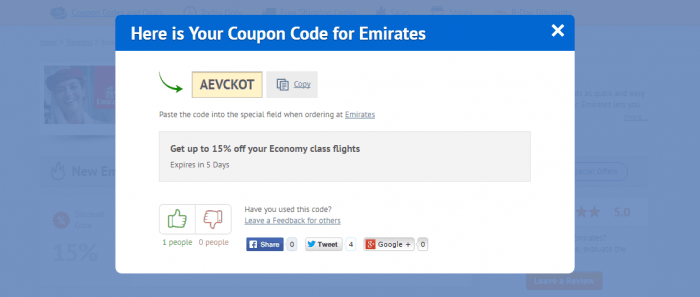The image depicts a website pop-up on a white background. At the top, there's a small blue banner with the text "Here Is Your Coupon Code for Emirates," with specific capitalization on the letters H, Y, C, C, and E. On the right side of this banner, there's an 'X' icon to close the pop-up.

Below the banner, a green arrow swoops down and points to the right towards a coupon code displayed on a light yellow background. The coupon code is "AEVCKOT," written in dark gray capital letters. Adjacent to the code is a small rectangular button labeled "Copy."

Further down, the instruction "Paste the code into the special field when ordering at Emirates" is displayed. This is followed by a gray banner that reads "Get up to 15% off your economy class flights." Underneath this, it states "Expires in five days."

At the bottom of the pop-up, there are thumbs up and thumbs down icons. One person has liked the post, while no one has disliked it. Additionally, there's a prompt that says "Have you used this code? Leave feedback for others." Below this, social media sharing options are available, with icons indicating that four people have shared it on Twitter.